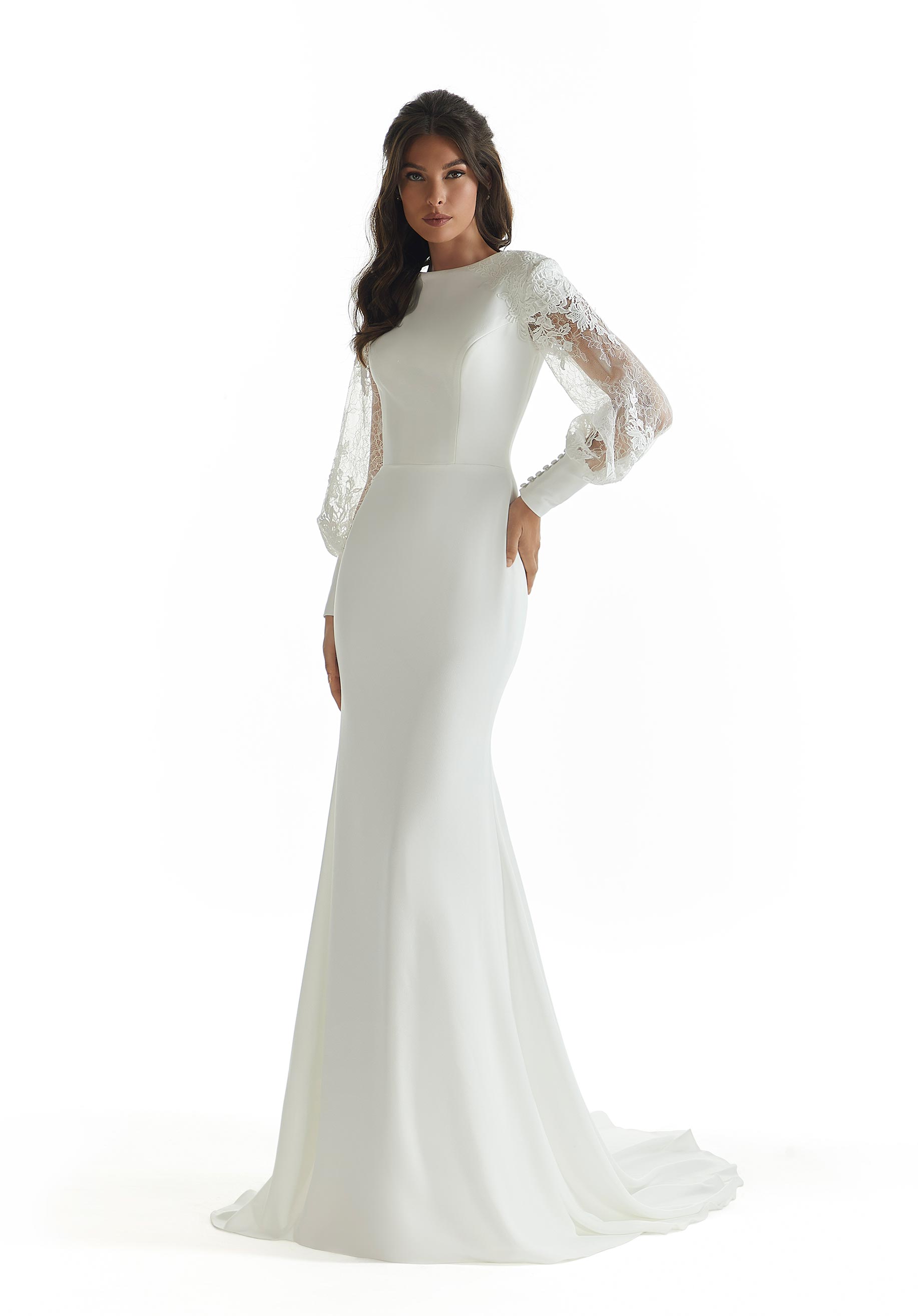This photograph features a striking young brunette woman with dark eyebrows and eyes, showcasing a wedding gown. She faces the viewer directly, posing gracefully with her left hand resting on her hip and her right hand hanging straight down. Her expression is neutral, imparting a serious look.

Her complexion is slightly tan, characterized as darker-skinned Caucasian. She is dressed in a long, form-fitting white gown that accentuates her hourglass figure, curving at the waist and hips before gently cascading to a small train on the ground. The dress, possibly from an advertisement, has long sleeves made of sheer lace material, which culminate at the wrists in solid white cuffs adorned with satin-covered buttons. The overall design is elegant yet understated, adding to the sophisticated appearance of the model. The background is completely white, ensuring that all attention remains on her and the gown. Additionally, there might be a hint of a veil tucked into her hair, flowing behind her.